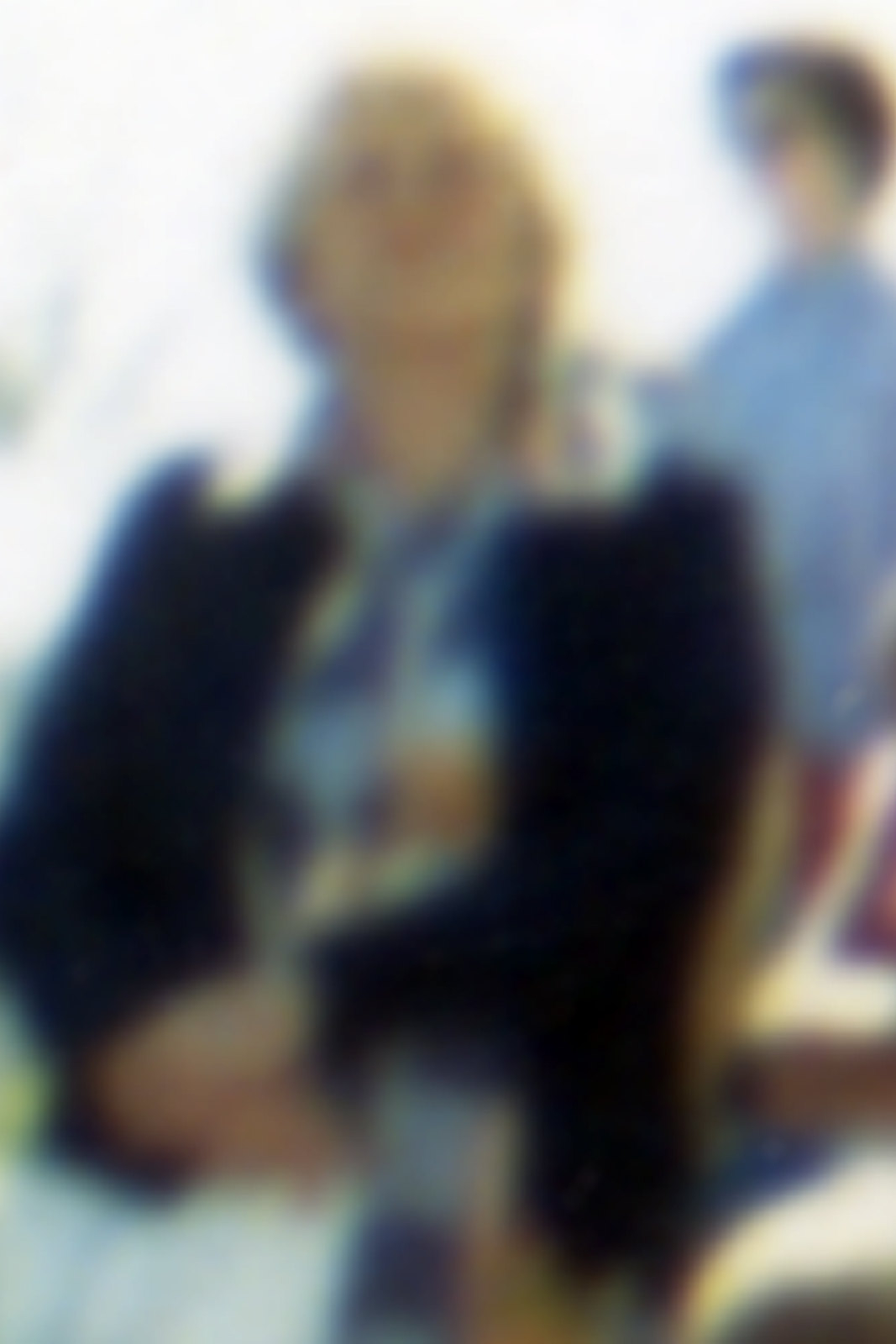In this blurry outdoor photograph, a middle-aged woman with short blonde hair and glasses stands under the sun. She is dressed in a stylish blue, white, and gold patterned blouse with a collar, layered with a navy blue cardigan sweater. She holds a white purse in her hand. Positioned behind her is another woman with short dark brown hair, also wearing glasses, dressed in a light blue blouse. They appear to be in front of a white backdrop, possibly a sheet or tent, suggesting the setting might be an outdoor event or gathering. The sunlight illuminates the scene, adding a warm, natural glow.